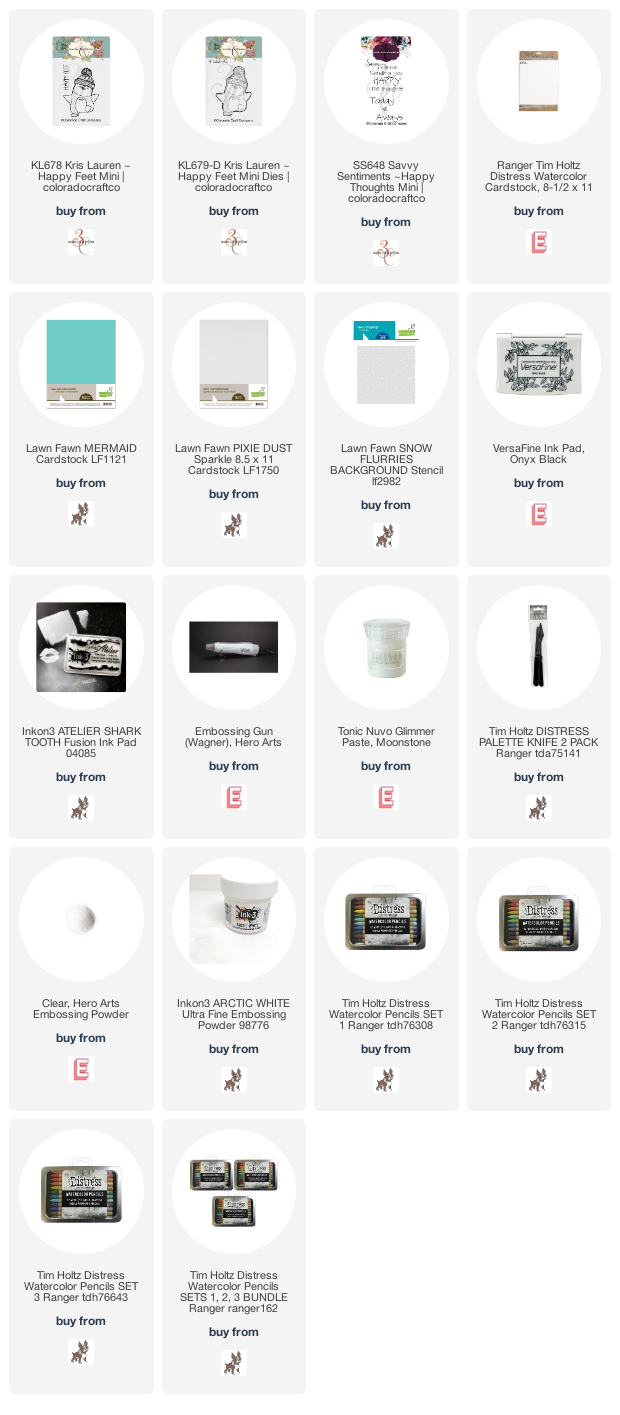The image showcases a selection of art and craft supplies available for purchase online. Featured prominently is the "Chris Lauren Happy Feet Mini," which appears to be an art book or similar creative item available from the retailer 3C. Alongside, an almost identical item, the "Chris Lauren Happy Feet Mini Dies," can also be purchased from 3C. Another similar product, the "Savvy Sentiments Happy Thoughts Mini," is listed under the same retailer.

Notably, the "Ranger Tim Holtz Distress Watercolor Cardstock" is available for purchase from a different retailer, indicated with an E logo. Additionally, the "Tim Holtz Distress Watercolor Pencil Set" is offered in individual packs or a three-pack option, broadening the choice for potential buyers.

All the items are visually represented in the image, showcasing their various types of packaging. These small, easily shippable items appear to be conveniently purchasable online, with the image suggesting a variety of retailers where these products can be found. The overall presentation emphasizes a curated selection of compact, user-friendly art supplies.